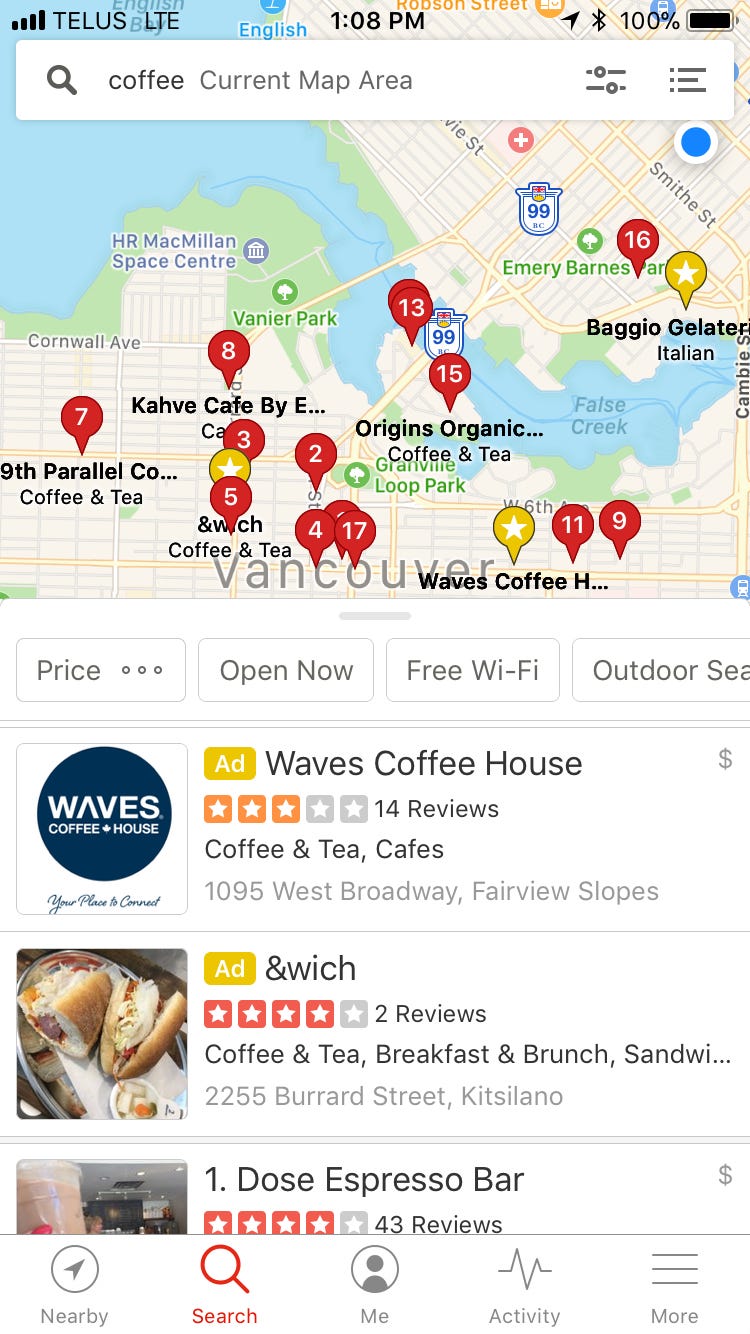The screenshot captures a Google Maps search on a smartphone at 1:08 PM, with the battery fully charged at 100%. The search bar at the top shows the word "coffee," indicating a search for coffee shops in the current map area. Below the search bar, a map highlights various coffee shop locations marked by red circles with numbers, suggesting the search is taking place in Vancouver.

Under the map, there are four filters available for refining the search results: price, open now, free Wi-Fi, and another filter that is mostly cut off but appears to indicate outdoor seating. 

Three specific coffee shop options are partially captured in the screenshot:

1. **Wave's Coffeehouse**: Listed with 14 reviews and classified under "coffee and teas, cafes." The address provided is 1095 West Broadway, Fairview Slopes.
   
2. **A partially visible coffee shop**: It shows an image of a sandwich and includes categories "coffee and tea," "breakfast and brunch," and "sandwiches." The address shown is 2255 Byrne Street, Kataslina, but the name is cut off.
   
3. **Dose Espresso Bar**: The entry displays part of an image, along with 43 reviews. 

The screenshot provides a quick snapshot of a user's attempt to locate a coffee shop in the area, complete with detailed search filters and a few options to consider.